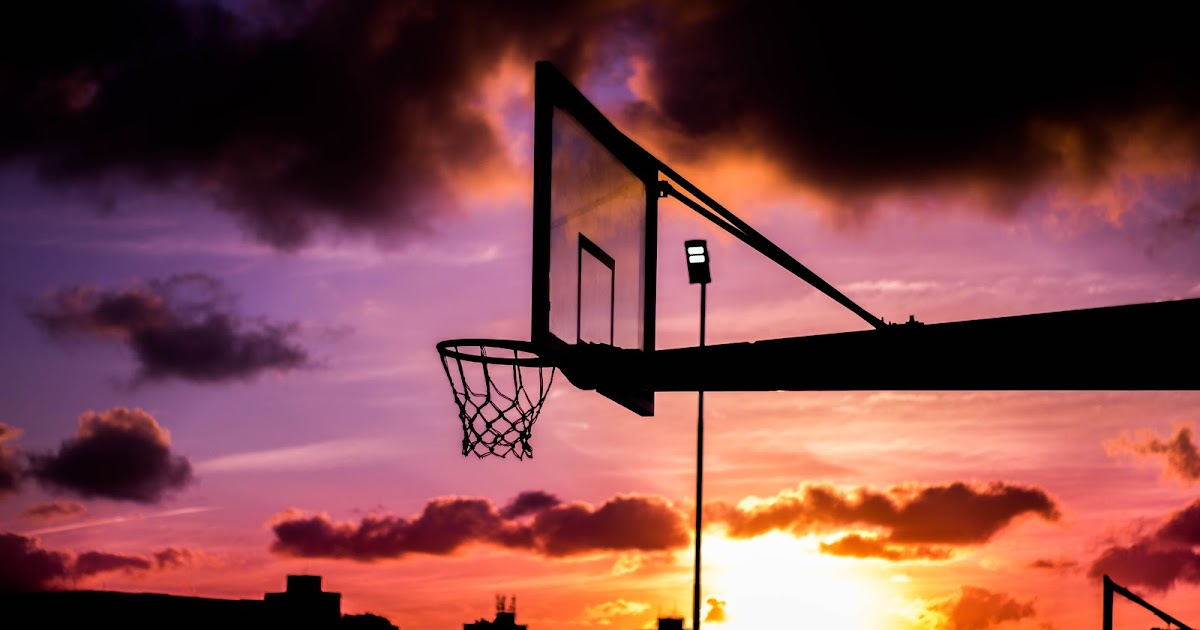The image captures a basketball hoop silhouetted against a vibrant sunset sky. In the center of the picture, a basketball net and backboard are prominently featured, with a large, horizontally extending stanchion that reaches out from the right center of the image. The sky behind the hoop transitions dramatically from purple to orange, streaked with white, and is filled with dark clouds in the upper left and right corners, as well as some black clouds on the left side. A modern LED street lamp rises from the base of the stanchion, illuminating the scene with a dim glow that highlights the court's details. The silhouetted outlines of buildings populate the lower left and center bottom of the frame, casting stark shadows against the vibrant, cloudy sky.